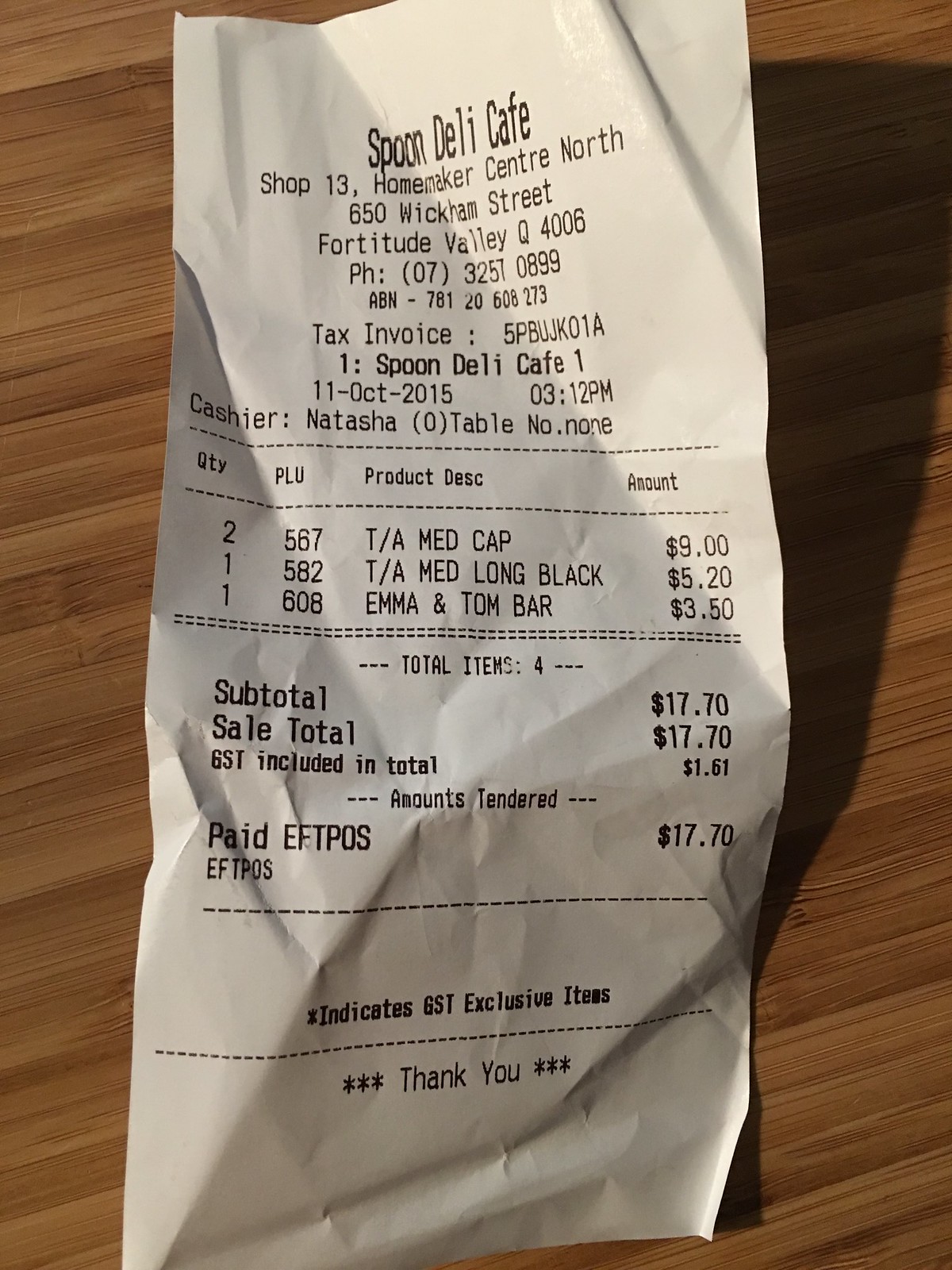This detailed photograph depicts a wrinkled and previously folded receipt from Spoon Deli Cafe, situated at Shop 13, Homeacres Centre North, 650 Wickham Street, Fortitude Valley, Q4006. The receipt, printed on white paper with black ink and placed on a brown table, itemizes an order processed by cashier Natasha on October 11, 2015, at 3:12 p.m. The items purchased include a medium cappuccino priced at $9.00, a medium long black coffee for $5.20, and an Emma and Tom bar for $3.50, amounting to a subtotal of $17.70. The total, inclusive of a GST of $1.87, remains $17.70, indicating the tax was incorporated in the subtotal. The receipt concludes with a "Thank you" note at the bottom, which, along with the details, portrays a typical dining transaction at the Spoon Deli Cafe.